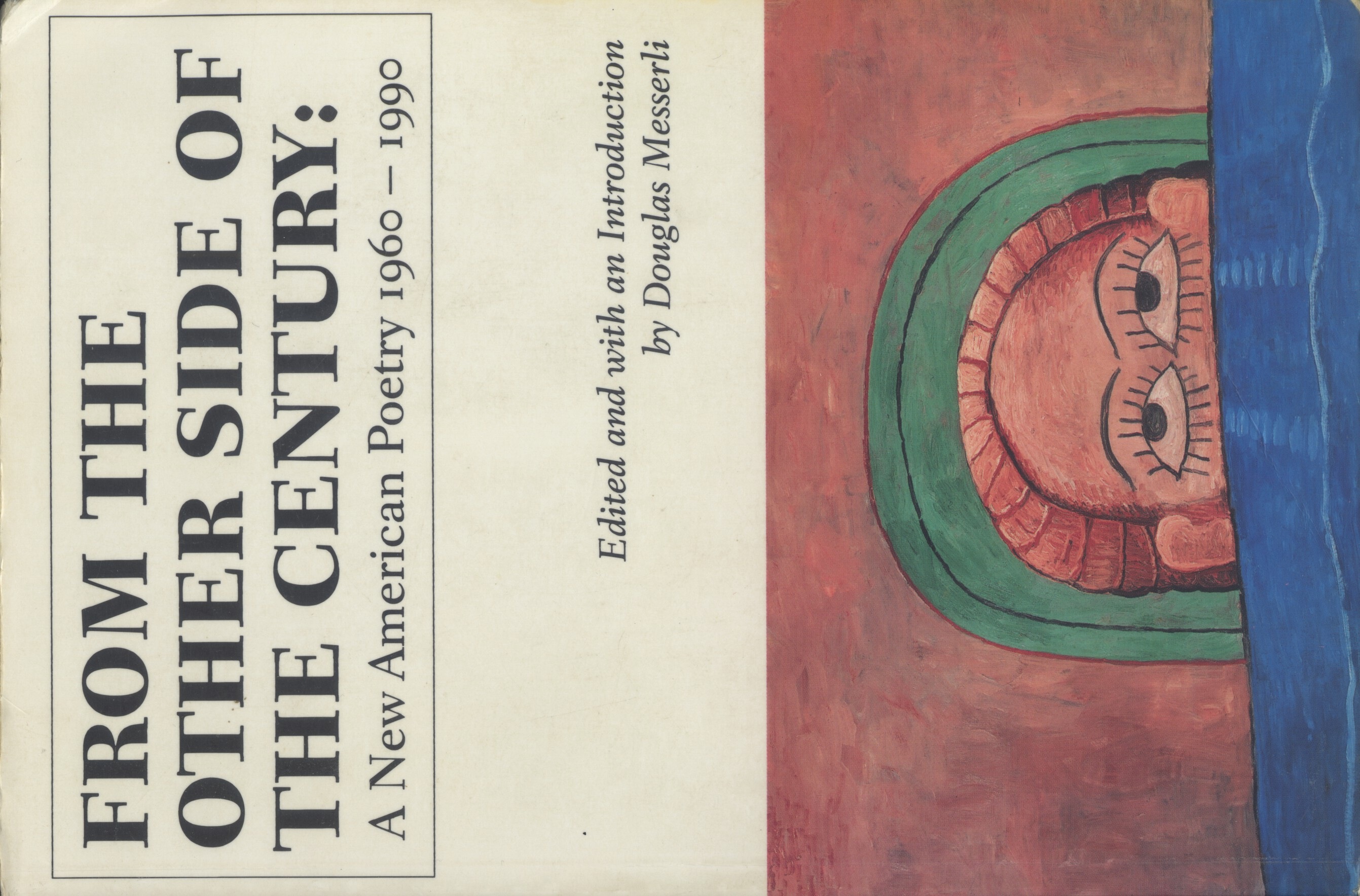This image is a photograph of a book cover, turned sideways, titled "From the Other Side of the Century: A New American Poetry, 1960 to 1990," edited and with an introduction by Douglas Messerli. The top half of the cover features the title in black and red lettering on a tan background, with the editor's name prominently displayed in black letters on a white background. The bottom half of the cover showcases a painting with a brown background, depicting a cartoonish, artistic image of a person's head peeking over the edge of a blue table. The individual has large, expressive eyes looking upward, brown hair, and either a green hat or a green halo-like arch behind them. The overall style of the drawing is simplistic and sketch-like, giving it a unique, amateurish charm.